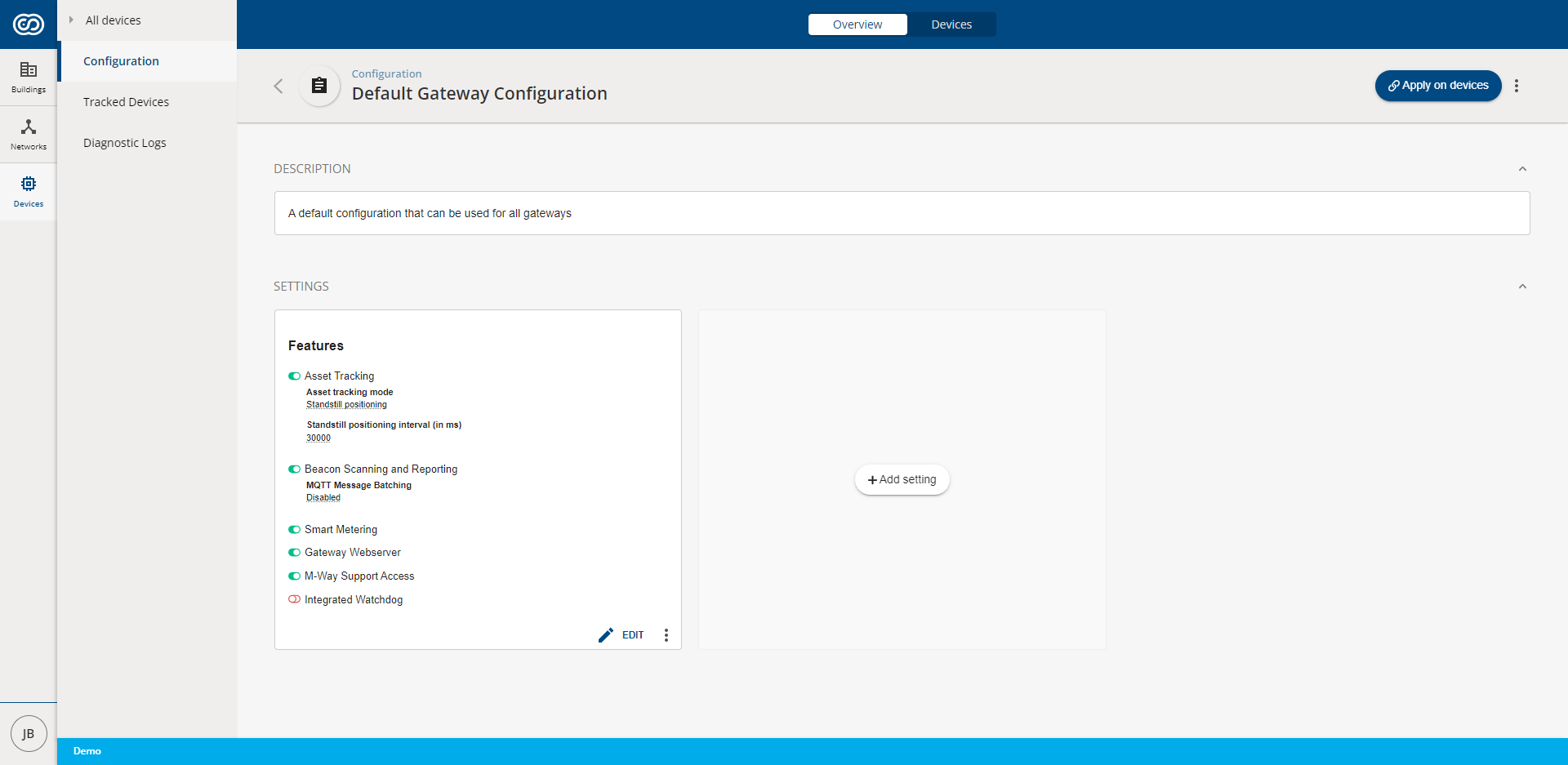The image displays a highly detailed user interface for a device management system. The layout comprises several distinct sections within a rectangular frame, described as follows:

Starting from the top left corner, there is a dark blue square featuring a white, horizontally-oriented 'S' logo. Adjacent to this square is a gray section labeled "All Devices." The remaining top bar is dark blue, containing a central white tab that says "Overview." Next to "Overview" is another tab labeled "Devices," written in a very light white font.

Directly beneath this top bar, the interface is organized into several columns. The first column starts with another "All Devices" label, followed by sections labeled "Configurations," "Track Devices," and "Diagnostic." There is an additional section whose label is partially obscured and difficult to read. 

Midway through the interface, another white square appears, titled "Features." Within this square, there is a subsection labeled "About Tracking," followed by a list of six bullet points. Each bullet point is accompanied by a green indicator, suggesting activation, except for the last one, which is turned off. At the bottom right of this white box, there is an "Edit" option accompanied by a pen icon.

To the far right of this interface, there is another box labeled "Add Settings," which seems to be a button or interactive element.

Overall, the design conveys a comprehensive and organized system for managing various device settings, configurations, and features.